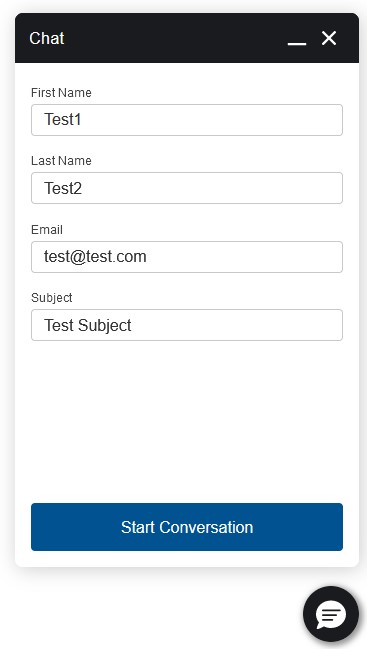The image is in portrait orientation, making it taller than it is wide. At the very top, a black banner spans from left to right. On the left side of the banner, the word "chat" is prominently displayed in white lettering. On the right side, there are two white icons: a horizontal line and an "X". 

Below the black banner, the image features four text fields on a white background. Each text field is preceded by a label and contains sample text:
1. The first text field is labeled "First Name" and contains the placeholder text "test one".
2. The second text field is labeled "Last Name" with the placeholder text "test two".
3. The third field is labeled "Email" and displays the placeholder text "test@test.com".
4. The fourth and final field is labeled "Subject" with the placeholder text "test subject".

At the bottom of these text fields, a conspicuous blue button extends from left to right. The button is labeled "Start Conversation" in white text. Below the blue button, a small black circle with a white speech bubble inside is visible. The speech bubble contains three black horizontal lines of decreasing length from top to bottom, symbolizing text or a chat function.

The setup suggests a form to initiate a chat session, probably with an online bot or support service. Users are required to input their first name, last name, email, and subject before clicking the "Start Conversation" button to begin the interaction. The exact nature of the chat is unclear, but it could be intended for customer support, inquiries, or feedback.